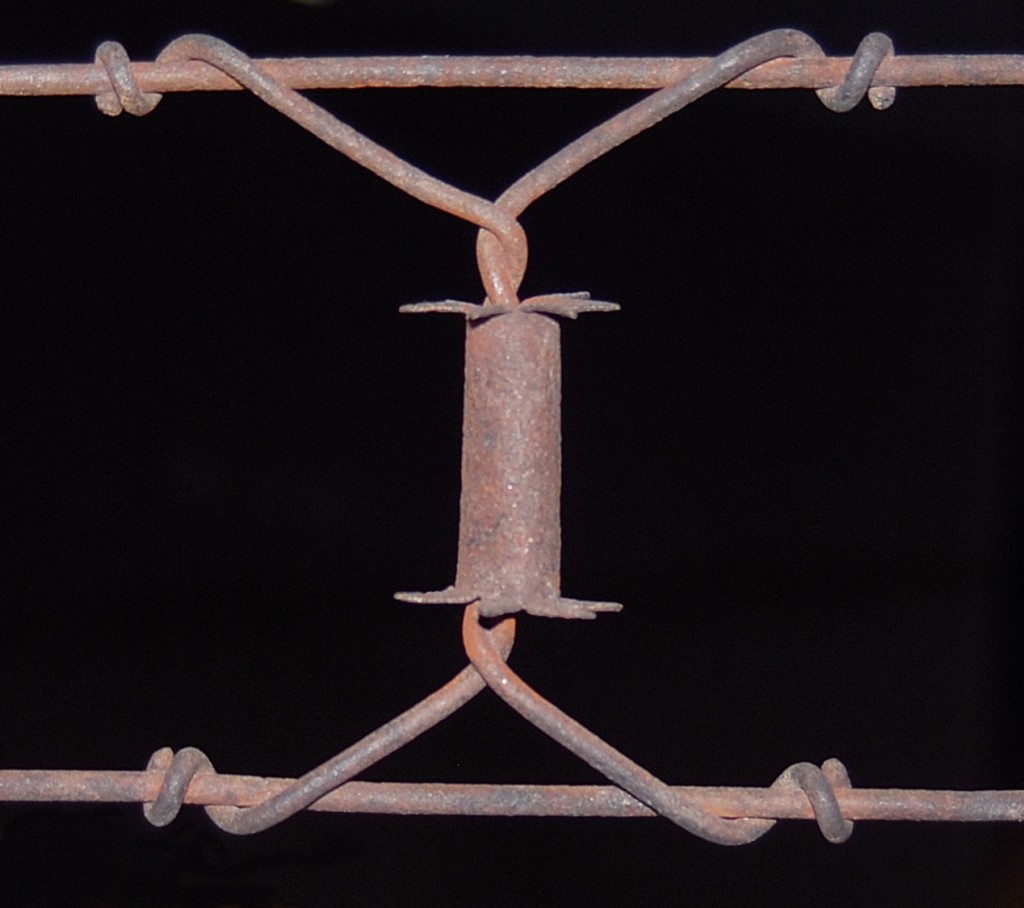This detailed photographic image captures a close-up of a rusty section of barbed wire, set against a dark, black or brown background. The composition features two horizontal wires that stretch from the left to the right edges of the frame, parallel to each other. Connecting these horizontal wires, at intervals, are twisted wires that form an X-shape with a central barbed cylinder. This cylinder, acting as the barb, has a series of spikes that could deter any attempt to breach the barrier. The twisted, Y-shaped wires knot around the top and bottom horizontal wires, securing the spiked cylinder firmly in place. The rust covering the wires and barbs attests to the age and weathering of this object, suggesting it may have once been used to contain livestock like cattle. The overall image is stark and evocative, emphasizing the menacing nature of the rusted barbs against the shadowy background.